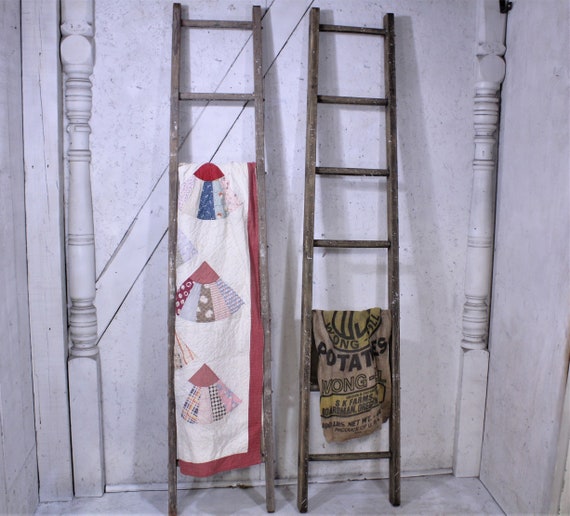The photograph captures an indoor scene featuring a narrow, white-walled space, approximately six feet wide, reminiscent of a small area such as the back of a closet. The wall is plain with no windows or doors, but two ornate wooden beams or columns frame the sides, carved with intricate spiral designs.

Against this minimalist backdrop, two tall, aged wooden ladders are leaned side by side in the center of the image. Each ladder is about seven feet tall with seven rungs, emphasizing their considerable height. The ladder on the left prominently displays a quilt draped from the third rung from the top. The quilt features a white base with a red border and patterns resembling quarter circles or hand fans made from various materials. On the right, the second ladder has an old potato sack hanging over the second and third rungs from the bottom. The sack is brown with silkscreened letters spelling out "POTATOES" prominently, and beneath that, the word "Wong", partially obscured by a fold. There also appears to be a logo above the text on the sack. These rustic elements against the plain background create a focus on the textures and details of the wooden ladders and their draped items.